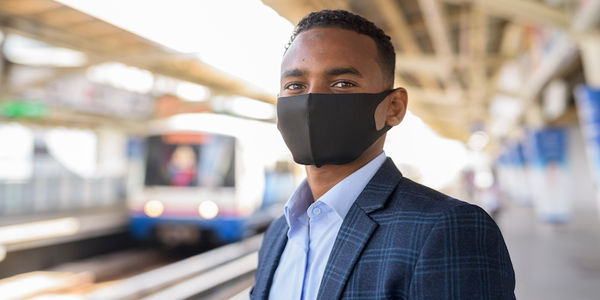In this image, a young man with dark skin, possibly of African or Middle Eastern descent, stands on an elevated train platform on a bright, sunny day. He is dressed in a sophisticated blue ensemble, featuring a light blue patterned checkered blazer over a blue dress shirt. His short hair is shaved on the sides, and he is wearing a black mask that covers his nose and mouth, indicative that the photo might have been taken during the COVID-19 pandemic. The blurred background reveals a train approaching the platform, with no other people visibly present, emphasizing the man's solitary presence as he waits to board. His gaze is directed at the camera, giving a poised and confident impression.